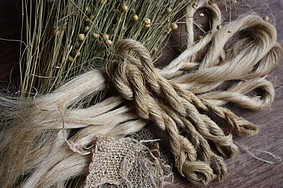In the image, there are intertwining strands of blonde hair and various ropes, creating a tangled, intricate display. These strands and ropes are layered atop one another on a surface that appears to be either a table or a floor, characterized by earthy brown and gray tones. Among the tangled materials, green strands resembling grass or weeds are also present, adding a touch of natural color to the scene. The scene seems almost sculptural, with hints of a wooden head form emerging from the knotted mass. Overall, the image’s color palette is dominated by yellows, browns, and greens, enhanced by a darker, filtered effect that gives it a subdued, moody atmosphere. The objects are densely packed, filling the entire frame with their complex, intertwined forms, as if carelessly laid together and captured from above.